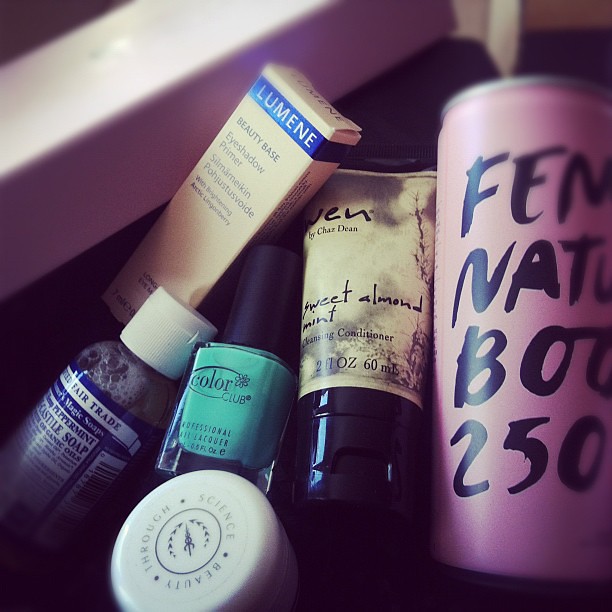This photograph captures an assortment of six beauty and facial products grouped together on a black surface, possibly a table. The setup includes a variety of containers arranged both horizontally and vertically. To the right, there's a pinkish can with partially visible black text reading "FEM NAT BOO 250," likely hinting at feminine or natural body care. Adjacent to it is a white tube labeled “Sweet Almond Mint” and “Cleansing Conditioner” with a black lid, marked as “Jen by Chaz Dean.” Moving left, you'll find a bluish-green nail polish with a black top. Above this, there is a cream-colored box indicating "Lumene Beauty Base Eyeshadow Primer" with a blue banner. Below the nail polish is a bottle containing a clear liquid labeled as "Fair Trade Magic Soaps." Lastly, there's a small canister with a lid that reads "Through Science Beauty." The background is somewhat indistinct but features a cream-colored box in the top left corner, which may be part of the setting.